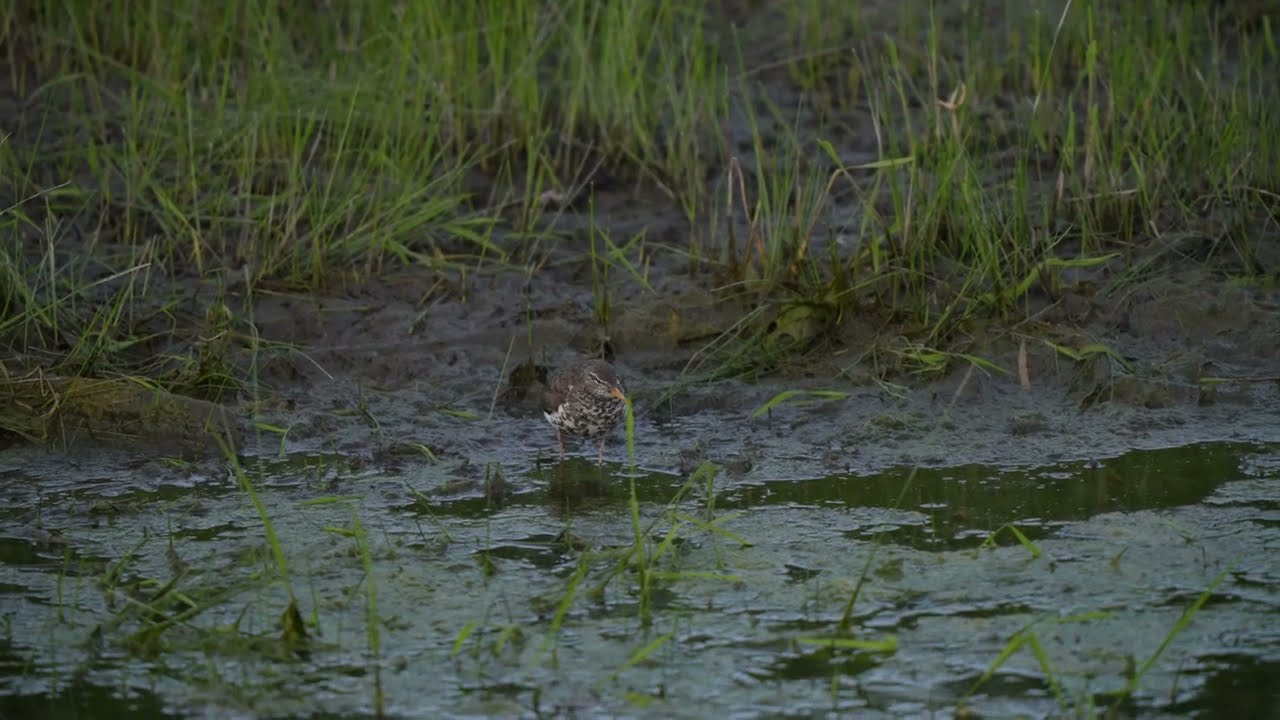The high-quality outdoor image depicts a side view of a swampy area. The top half of the image features a muddy shore with sparse but long-bladed grass clumps interspersed with patches of short green and dead brown grass. The mud appears thick and wet, creating a soupy, squishy texture. Dominating the bottom half of the picture is a body of stagnant, dark green water filled with thick algae, giving it a murky appearance. Bits of tall green grass poke through the water, which is otherwise around 80% covered by the floating green algae. At the center of the image, a small brown and white speckled bird stands ankle-deep in the water. The bird has short orange legs, a short orangish-yellow beak, and distinct black eyebrows framing its black eyes. Its body is positioned at an angle, with its head slightly turned to the right, appearing to look forward.